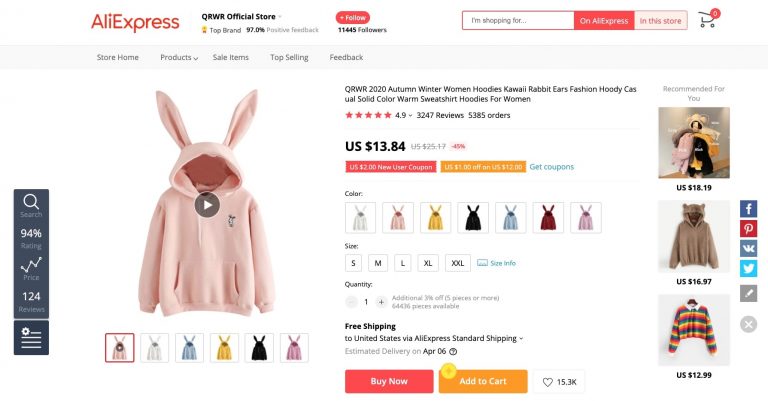The image captures a detailed view of a product listing page on Aliexpress, specifically for the "QRWR Official Store." The layout is left-to-right horizontal, suitable for browsing on a computer or smart device. The background primarily uses a plain white screen for clarity.

At the top left corner, the Aliexpress logo is prominently displayed. To the right of the logo, the text "QRWR Official Store" appears in black, accompanied by a small icon indicating it as a "Top Brand" with 97% positive feedback. A red "Follow" button with white text is situated next to this, showing that the store has 11,645 followers beneath it.

A white search bar is positioned towards the right side of the header, with the placeholder text "I'm shopping for..." Users can refine their search to either "on Aliexpress" or "in the store" via options next to the search bar. A shopping cart icon is also present, currently showing zero items.

Below the header, a gray horizontal menu bar provides quick access to different sections of the store, including "Store Home," "Products," "Sale Items," "Top Selling," and "Feedback."

On the right-hand side, a vertical gray rectangular section includes various interactive elements: a search magnifying glass icon, a 90% rating indicator, a price tracker with a zigzag line, 124 reviews, and settings options. Additionally, there's an image of a pink sweatshirt featuring bunny ears, with options to select different colors.

In the middle section, the product details are highlighted. The sweatshirt has a 4.9-star rating based on 3,247 reviews and a total of 5,385 orders. The price is prominently displayed, along with options to access US-specific coupons. Users can select the color, size, and quantity, with free shipping available. There are buttons for "Buy Now" or "Add to Cart," and users can "heart" the item, which already has 15.3k likes.

Along the right side of the page, recommendations for related products are provided. Further to the right, social media icons are available for easy sharing.